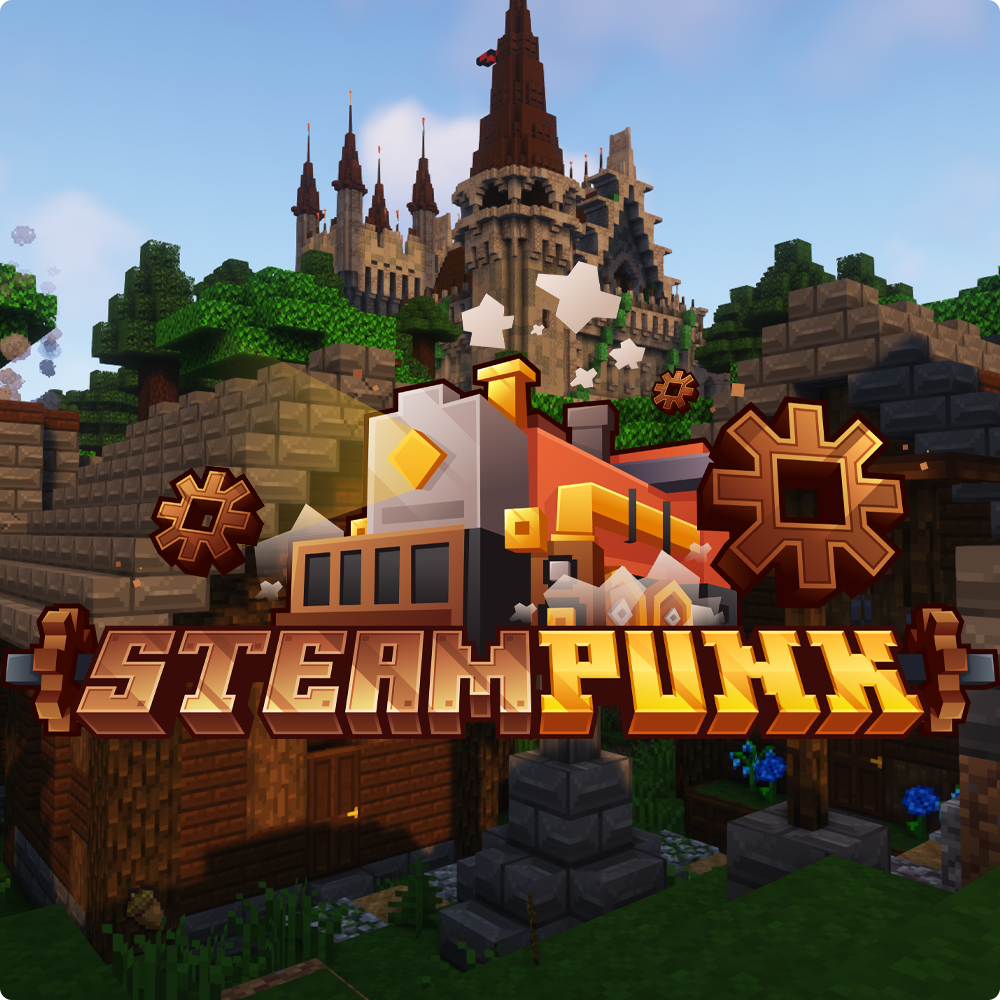The image is a square with subtly rounded corners, presenting a detailed, promotional scene from a video game inspired by Minecraft, titled "Steampunk." Dominating the center is a playful, stylish title with the word "Steampunk" split; "Steam" is in a copper-brown hue, while "Punk" is golden-yellow. Above the title, there are intricate steampunk gears and a small, Lego-like depiction of a train or building with chimneys, colored in shades of brown, black, orange, yellow, and gray.

In the background, the scenery is blocky and pixelated, featuring a castle with reddish-brown, pointed roofs on its towers. The castle, made up of brownish-gray blocks, stands amidst lush greenery composed of tall, blocky trees. The sky is a light blue with a few scattered clouds. Below the castle and trees, the foreground highlights a stone-roofed cabin-like structure set in a cavern environment, adorned with patches of blocky grass and flowers. The overall dark-to-light gradient from bottom to top enhances the depth and charm of this meticulously crafted steampunk world.